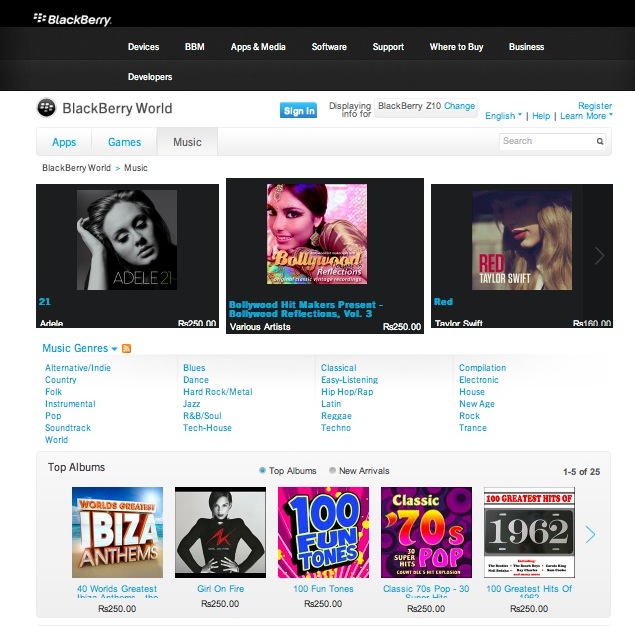This screenshot captures the homepage of a BlackBerry website. The top of the page features a dark white bezel with many dots on the left, followed by the bold white text "BlackBerry." Below this bezel is an off-gray rectangle with bold white tabs for navigation: Devices, BBM, Apps and Media, Software, Support, Where to Buy, and Business. 

Beneath another dark gray rectangle, the bold white text reads "Developers." In the main white area of the page, a black circle is present, containing numerous white dots. Adjacent to this circle, "BlackBerry World" is written in bold black text. On the far right, a cyan blue rectangle displays the text "Sign In" in white. Outside of this, black text states "Displaying Info 4," followed by another off-gray rectangle where "BlackBerry Z10" is written in black, and the word "Change" is highlighted in blue.

Further down, tabs for language selection, such as English, are available in hyperlink blue text, followed by black lines separating "Help," "Learn More," and "Register," also in blue text. Above these options are multiple selectable squares. The section title "BlackBerry World" appears in black, with a blue right-pointing arrow next to "Music."

Highlighted are three album covers. The first features a black and white photo of Adele, labeled "Adele 21" in white below her image. The text "21" is in bold blue, with "Adele" underneath in white. Both are priced at RS-250. Next, there is a Bollywood album cover portraying an Indian woman adorned with golden earrings, a golden clasp in her black hair, and a golden robe. Underneath, it reads "Bollywood Reflections" in gold and white text, with detailed descriptions and an RS-250 price tag. Finally, Taylor Swift's partial profile is seen with her signature red lipstick. "Red" and "Taylor Swift" are displayed in bold white and blue text, priced at RS-160.

At the bottom, there are multiple hyperlinks for music genres listed alphabetically, ranging from Alternative/Indie to Trance, encompassing genres like Country, Folk, Pop, Soundtrack, Retro, Blues, Hard Rock/Metal, Jazz, R&B/Soul, Tech House, Classical, Easy Listening, Hip Hop/Rap, Latin, Reggae, Techno, Compilation, Electronic, House, New Age, Rock, and Trance.